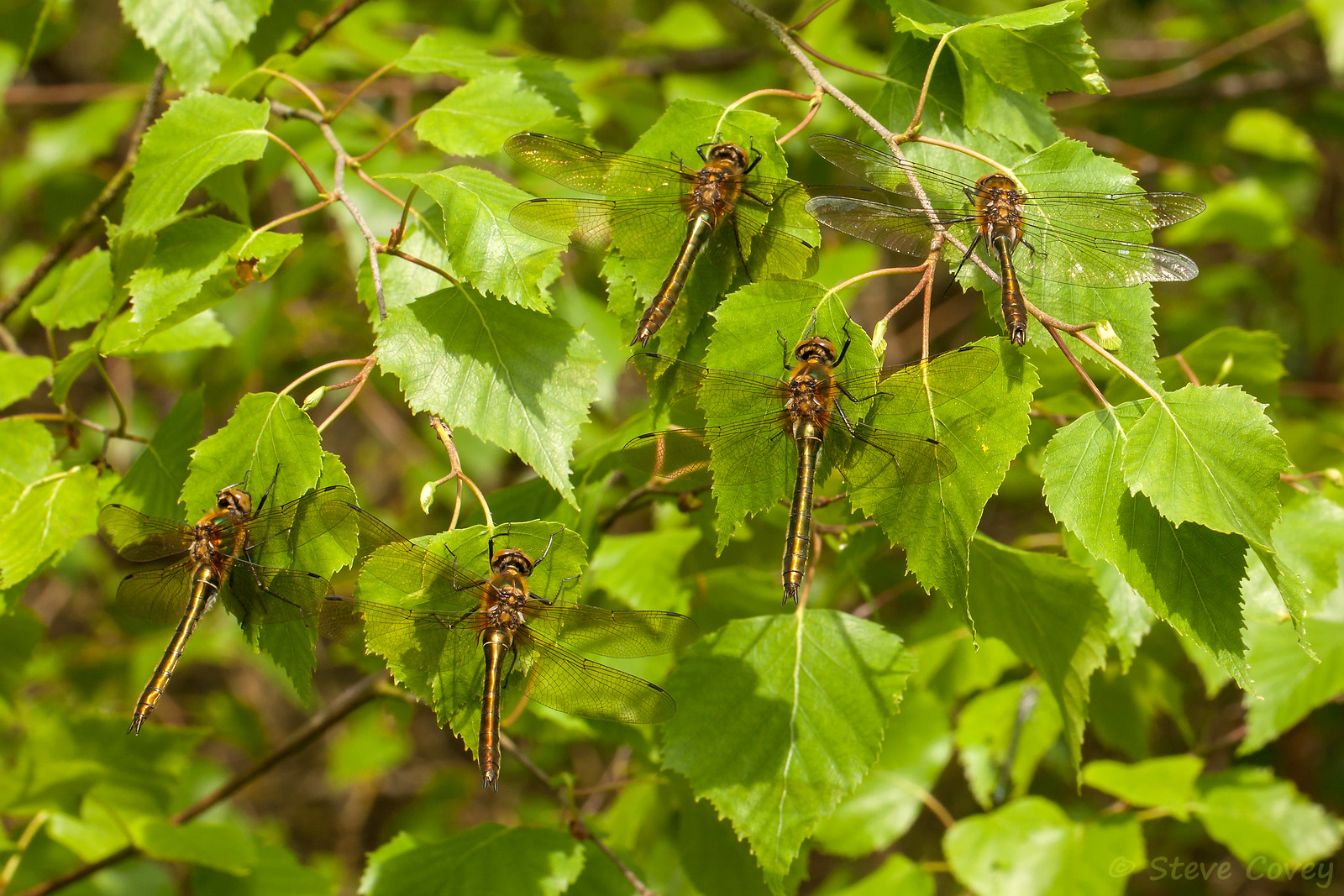The photograph captures a detailed close-up of a sunlit bush outdoors, featuring delicate teardrop-shaped leaves with serrated edges and intricate veins running from the central vein to the edges. The leaves exude a light green hue and are attached to thin twigs. Prominently inhabiting this vibrant greenery are five dragonflies, each with four translucent wings and iridescent greenish metallic abdomens, tapering to brown tips. Their long, slender tails add to their distinctive appearance. The dragonflies are strategically positioned around the image: two on the lower part, one in the center, and two directly above it, all facing away from the camera. The background reveals a blur of additional leaves and branches, enhancing the depth and natural ambiance of the scene. Notably, the bottom right corner features the faded gray text "Steve Covey," identifying the photographer or perhaps a title for the piece.